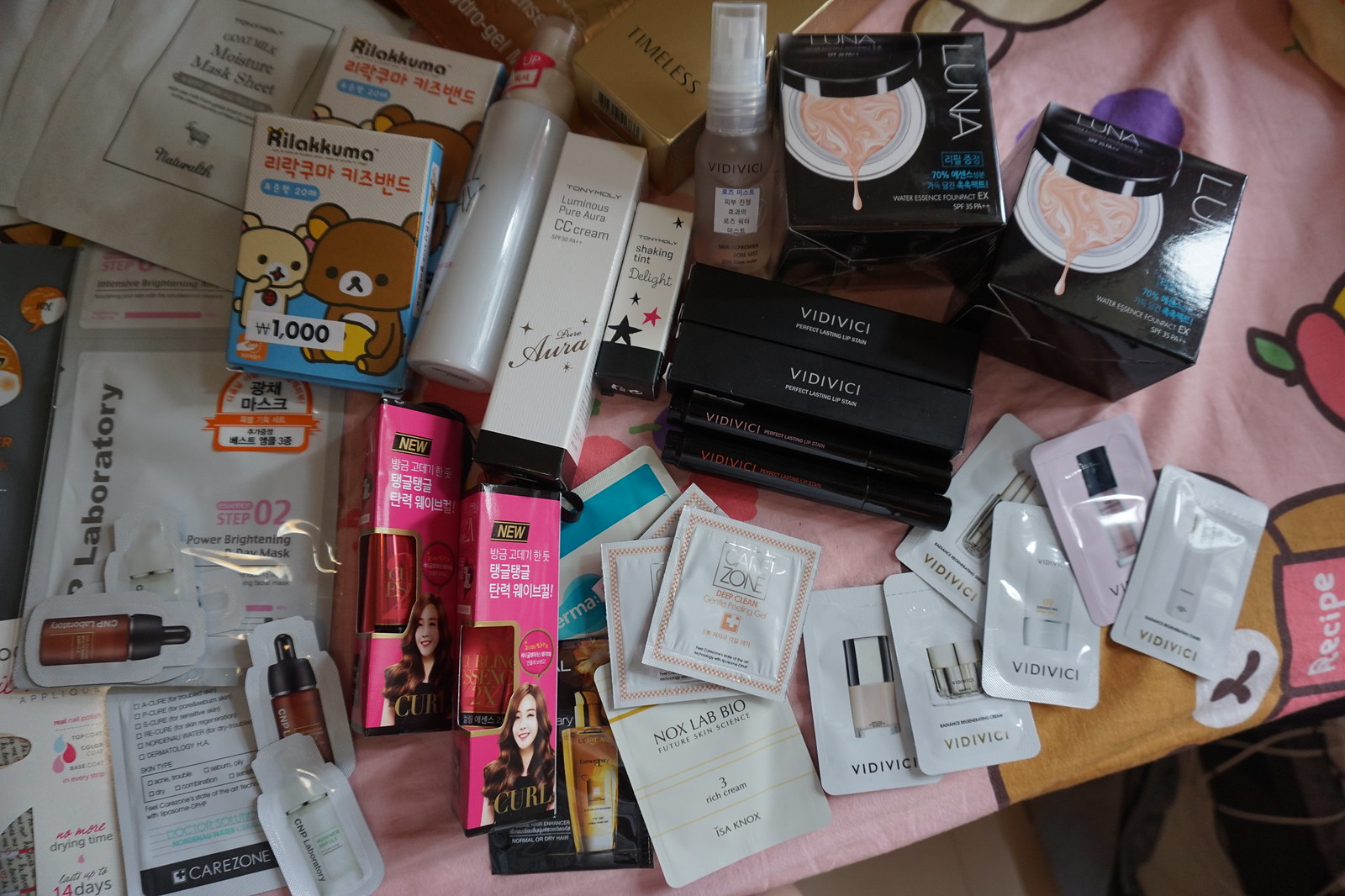The photograph captures a vividly colored scene centered around a surface covered with a tablecloth featuring shades of pink, green, and hints of brown. The table is adorned with a variety of cosmetic samples, resembling those typically found at a perfume counter. Among these samples are several white bottles, indicative of various skincare or makeup items. Prominently displayed are cosmetic products from a brand called Fitty Fizzy. Also present are sleek black boxes labeled "Luna" in white text, which contain foundation products. The boxes reveal the foundation in a pale pink hue, with a drop of the product visibly emerging from one of the bottles. Adding to the array, there are pink boxes likely containing lipsticks, distinguished by the clear tubes visible within and their pink accents. Overall, the table is a showcase of assorted beauty products, arranged to intrigue and captivate those with an interest in cosmetics.